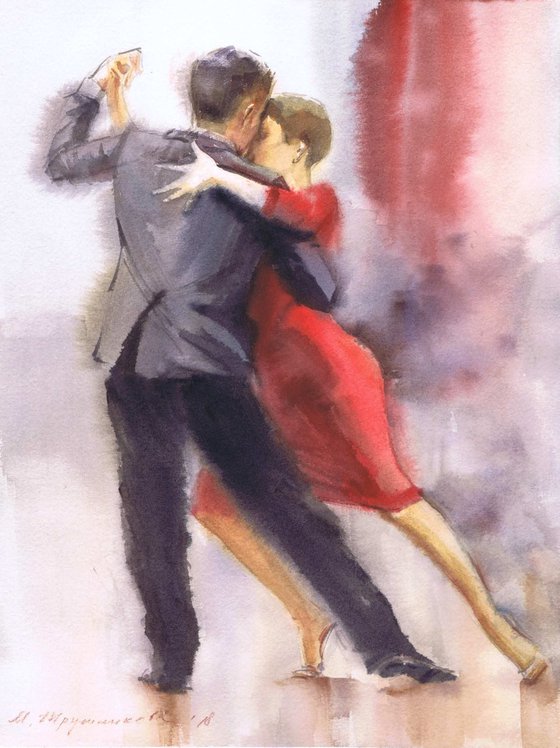This detailed watercolor painting captures a man and woman engaged in a dance, possibly the tango, against a nondescript, abstract background with shades of purple, red, white, and beige. The man, positioned on the left, is wearing a dark (possibly black or gray) suit and has medium-length black hair. He stands on his right toe, with his right leg extended to the side, while his left leg remains straight. His back faces the viewer, but his head is turned slightly to the right. He holds the woman with his right arm around her waist and his left hand clasping her right hand, which is raised.

The woman, situated slightly to the man's right, is dressed in a knee-length red dress and has short brown hair, adorned with an earring. She leans into the man, resting her forehead on his cheek, and gazes leftward. Her left arm drapes around the man's upper back. In her dance pose, she stands on her right toe, with her right leg bent at the knee and her left leg extended to the side, her foot angled outward. The background is an abstract blend of colors without any distinguishable objects, transitioning from light shades at the top to varying tones of purple and white in the middle, and brown and white at the bottom. A small, unreadable signature is located in the bottom left corner of the painting.